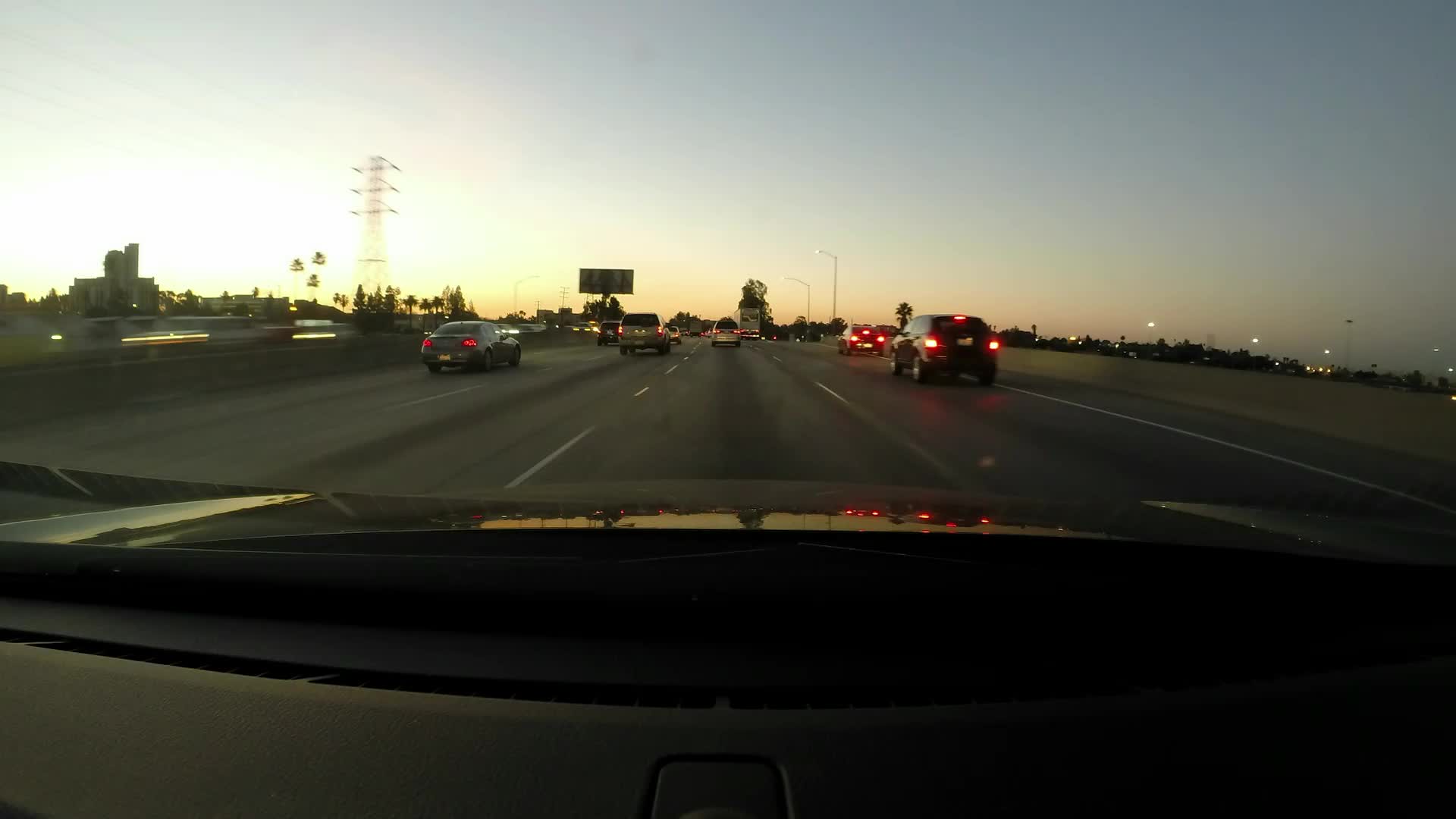A bustling multi-lane highway stretches out ahead with four to five lanes packed with vehicles, including several large tractor trailers. A solid barrier separates the lanes, with cars streaming in the opposite direction on the other side. A prominent cell tower stands tall amidst the scene, surrounded by numerous trees and other roadside elements. The sun is nearing the horizon, casting a golden hue across the landscape, indicative of rush hour traffic. On the right side of the road, a large billboard is visible. Tall streetlights line the highway, illuminating the path as twilight approaches. The perspective of the image is from inside a black car, with only the hood visible in the foreground, giving the viewer a sense of looking out through the windshield onto this vast, busy highway.